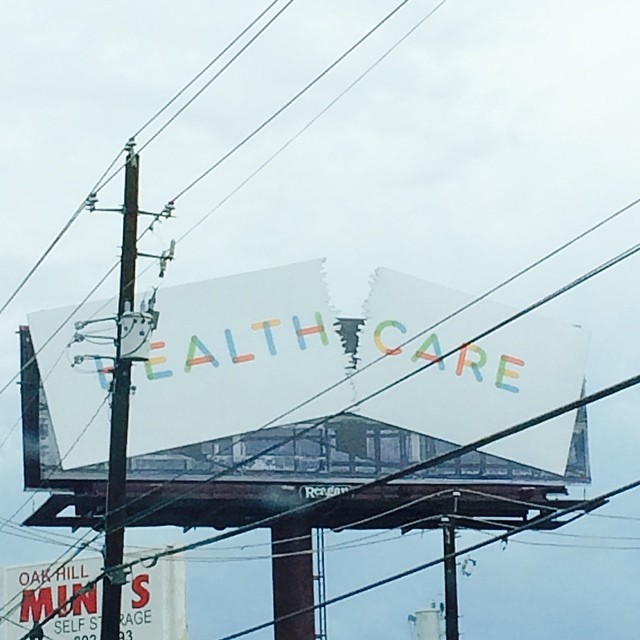The image depicts an upward view of a weathered billboard set against a backdrop of urban infrastructure. The billboard's message, intended to read "health care," is disrupted by a conspicuous tear down its center. The word "health" is displayed on the left segment, its letters vibrantly colored in red, yellow, green, and blue, set against a black background framed by exposed structural bars. The right segment, with a white background, bears the word "care," completing the intended message albeit in a fragmented form.

Prominent within the scene is a large telephone pole situated to the left of the billboard, adorned with an intricate network of wires stretching across the top, middle, and bottom portions of the image. In the background, a vast white water tank looms, adding depth to the urban landscape. Additionally, another billboard is visible to the left, characterized by its stark white background and bold red text advertising "Oak Hill Mini Self-Storage." The interplay of torn advertising and surrounding elements conveys a sense of industrial ambiance intertwined with the remnants of past promotions.